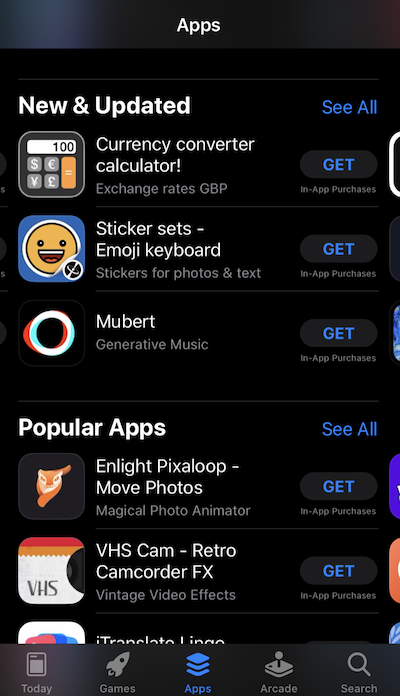This image is a screenshot displaying a section of an app store. At the top of the screen, there is a heading labeled "Apps," followed by a subheading that reads "New and Updated." On the right side of this subheading is an option to "See All." 

The first featured app is a "Currency Converter" which includes functionalities such as calculator, exchange rates, GBP conversion, and more. The second app is titled "Sticker Sets," offering emoji and keyboard stickers for photos and text customization. 

Next is "Mubert," an app focused on generative music. Below these apps, there is a section titled "Popular Apps." The first in this category is "Pixaloop," which is described as an English version, with features for animating photos and creating magical photo animations. Following it is "VHS Cam,” an app providing retro-themed video effects including Coda, FX, and vintage video styles.

At the bottom is the toolbar featuring options like "Today," "Games," "Apps," "Arcade," and a "Search" function, marking the end of the screenshot.